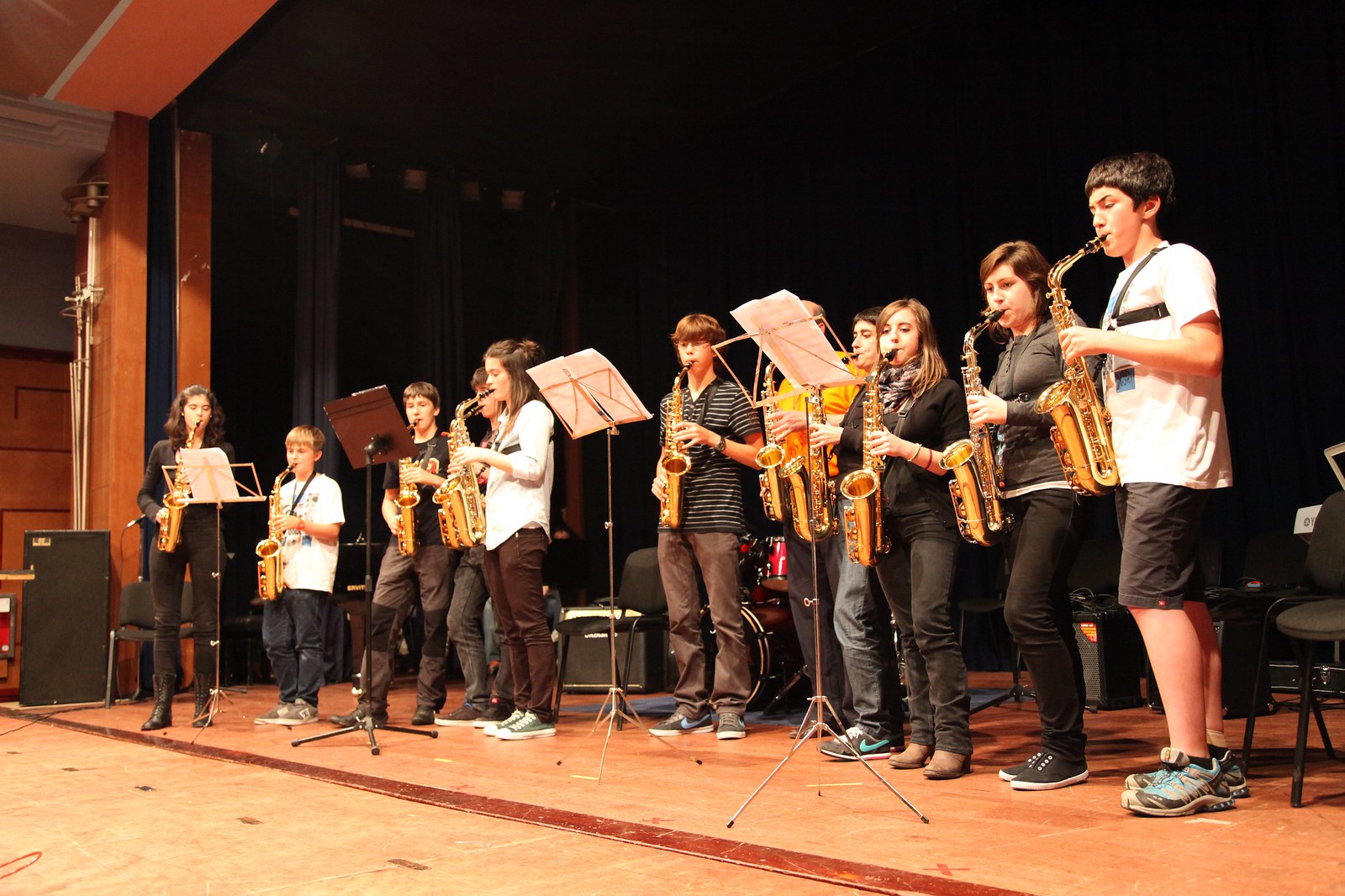The image captures a band practice or performance featuring predominantly saxophone players on a stage with light brown wooden flooring. The group comprises a mix of boys and girls, as well as one adult female who appears to be the instructor. The ensemble, which includes about 11 to 12 individuals, is organized in a row, attentively playing their golden saxophones. In front of them are four music stands displaying sheet music. Their attire is casual, consisting of hoodies, t-shirts, jeans, and trousers, with one person notably wearing shorts. Sneakers are the common footwear among them. Behind the group, a series of black chairs and various sound equipment, including amplifiers and a drum set, can be seen. The backdrop is a dark curtain with a few visible folds, contributing to a dimly lit stage ambiance. To the left side of the stage, there's a black speaker, and a piano is situated in the corner.